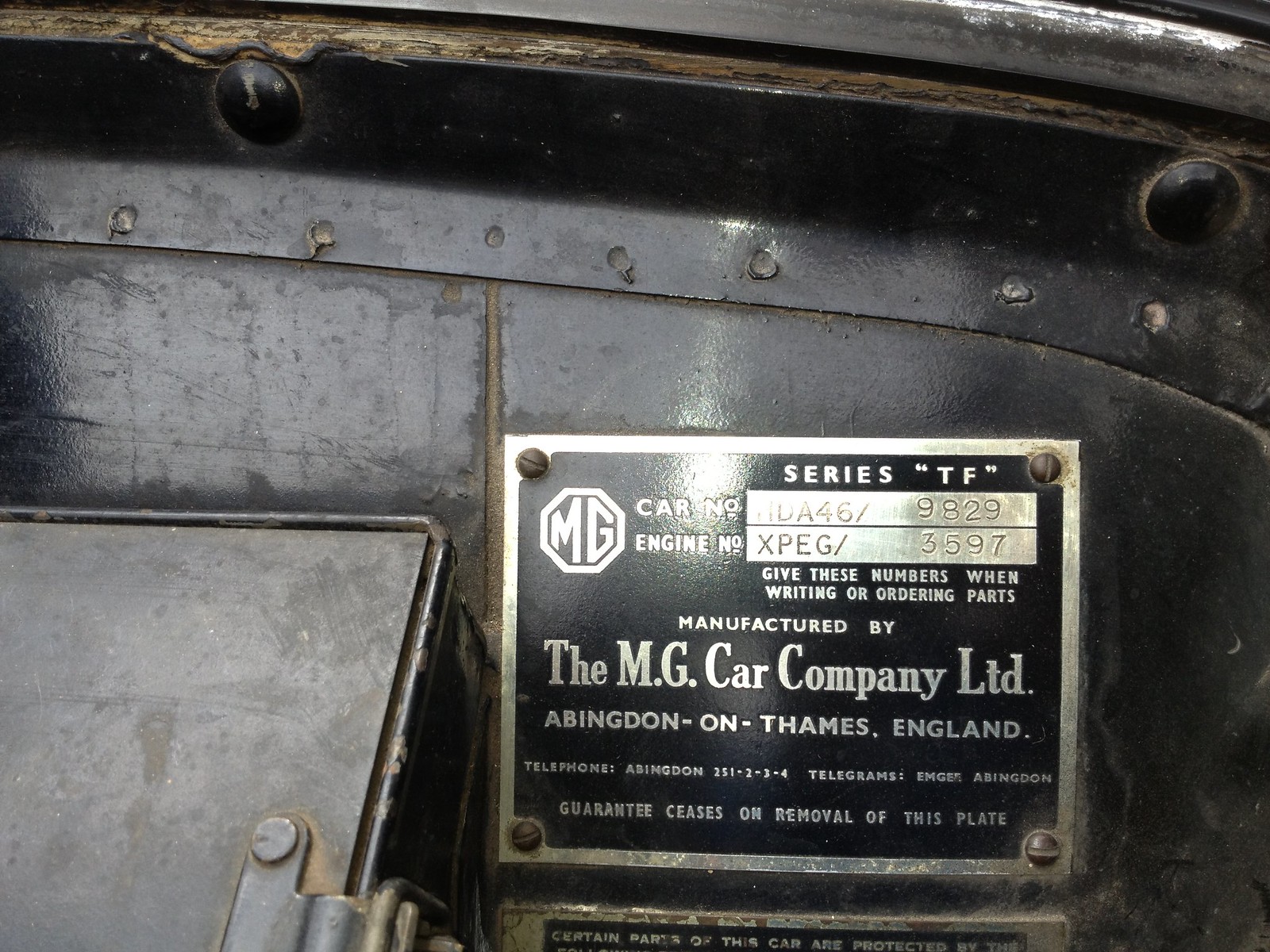The image captures a vintage MG car's engine bay, featuring a detailed metal identification plate on the firewall. This black and silver plaque displays essential information about the vehicle, including the "Series TF" model designation and specific manufacturing details. In the upper left corner, the MG logo is visible, while to the right, the car number "DA469829" and the engine number "XPEG3597" are prominently listed. The plate advises, "Give these numbers when writing or ordering parts," and the text further indicates that the car was "Manufactured by the MG Car Company Limited, Abingdon-on-Thames, England." Contact details, including a telephone number and a telegram name, are also provided. The plate is secured by four dark screws, one at each corner, and ends with a notification: "Guarantee ceases on removal of this plate." The overall condition of the plate and the car's interior suggests that it is a classic or vintage model.